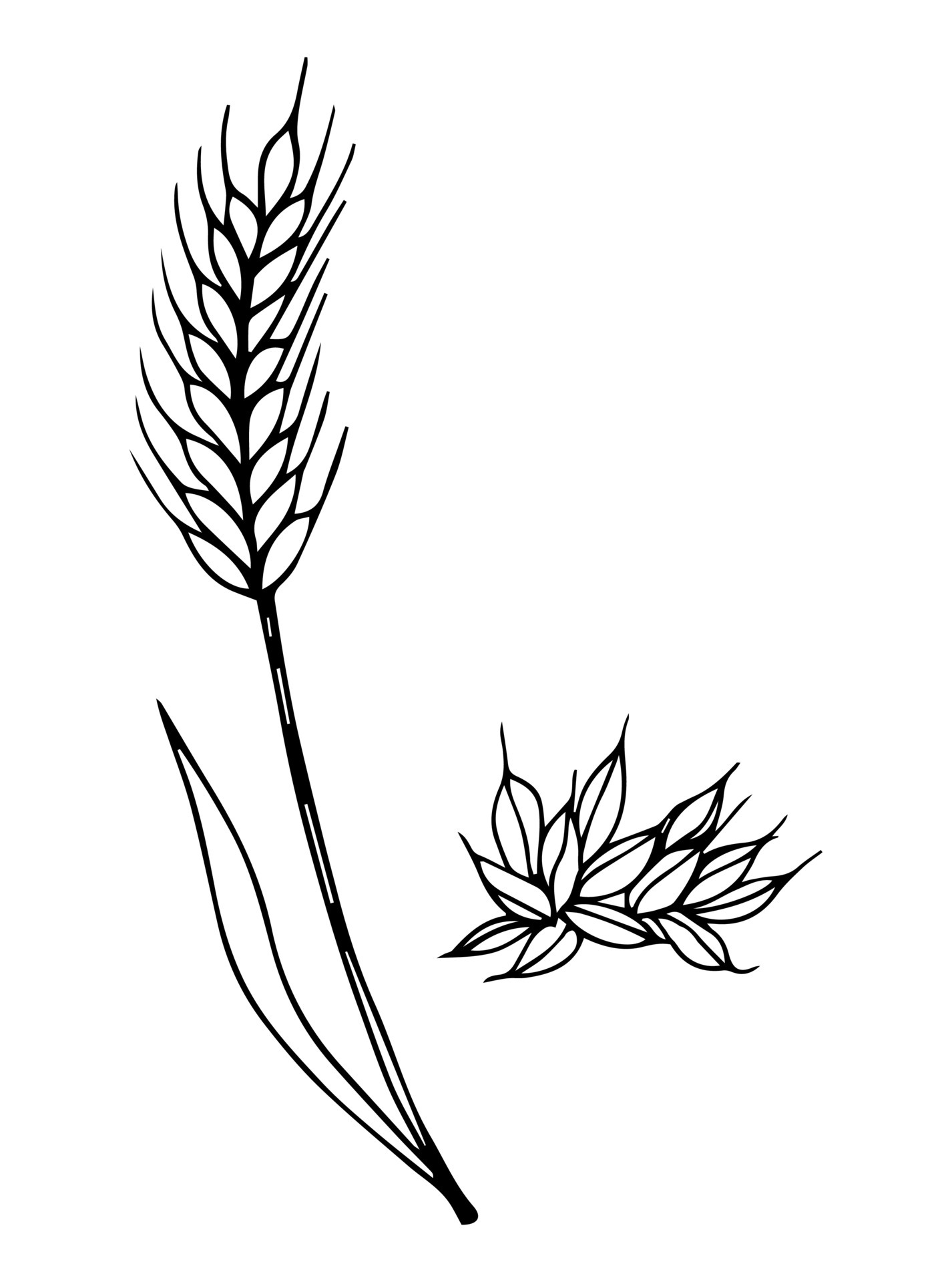In this image, a simplistic yet meticulous black ink sketch of a wheat plant is depicted against a solid white background, which dominates the composition. The artwork features a prominent single stalk of wheat positioned on the left-hand side, reaching upwards with a long, thin leaf growing from the stem and coming to a sharp point. Notably, this singular leaf lacks intricate details such as spines or veins, being rendered as a plain outline. Towards the bottom right-hand side of the image, there is a clustering of ovular wheat kernels, each characterized by long, delicate hairs, resembling the top of the wheat stalk. This sketch captures the essence of the wheat plant with minimalistic black lines and outlines, emphasizing both the structure of the wheat stalk and the scattered kernels beside it.